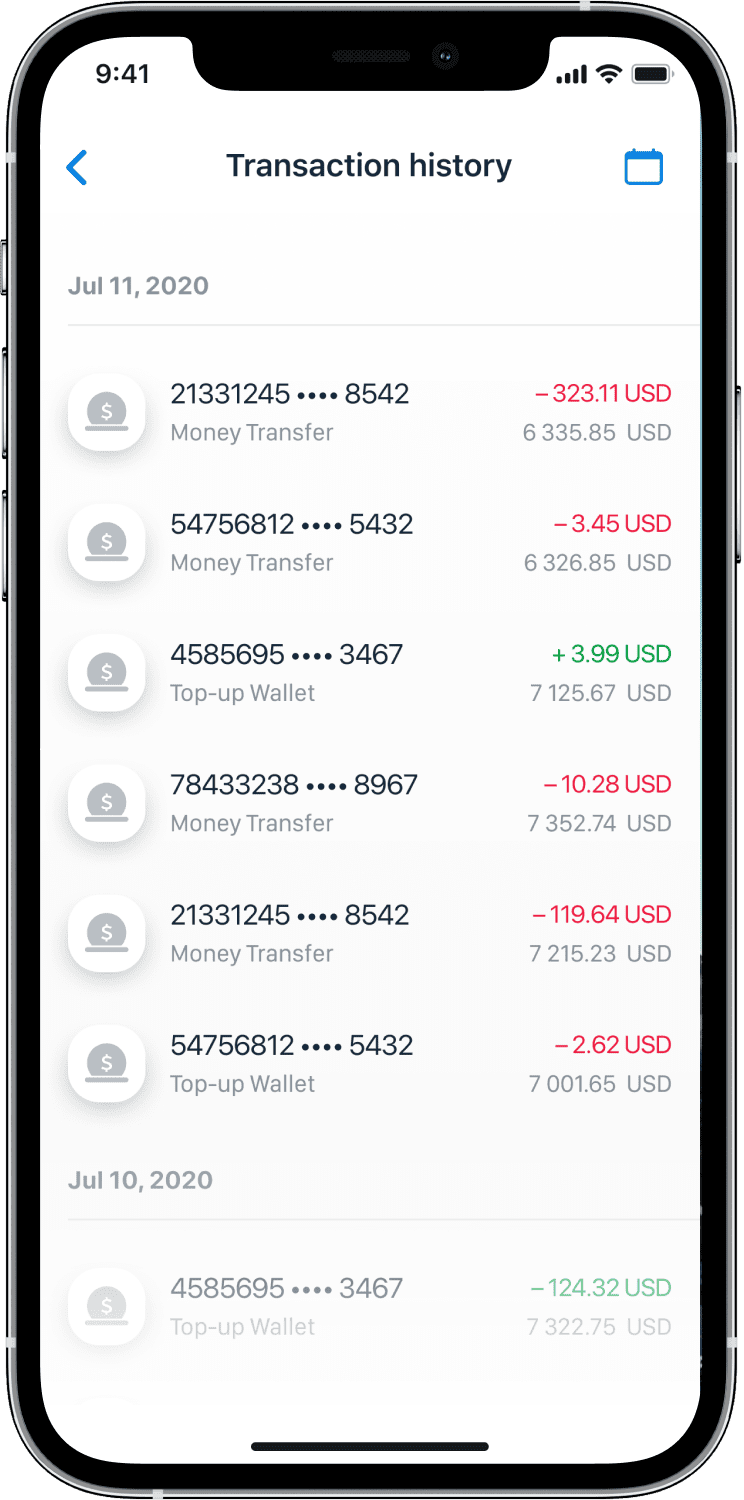A photograph captures the transaction history displayed on a cell phone screen, which is encased in a black cover. The phone screen, predominantly white, shows various details. At the top left, the time reads "9:41," while the top right corner displays Wi-Fi, battery, and data connectivity symbols. The main heading reads "Transaction History" followed by the date "July 11, 2020."

Below the date, various transactions are listed:

1. The first two entries are labeled "Money Transfer".
2. The third entry is labeled "Top-up Wallet".
3. The fourth and fifth entries are also "Money Transfer".
4. The sixth entry repeats "Top-up Wallet".

Listing below "July 10, 2020," another entry indicates a "Top-up Wallet" transaction, followed by several transactions characterized by their numerical changes.

To the left of "Transaction History," a blue arrow button points left, and to the right, there is a blue icon resembling a calendar or box.

The transactions are color-coded: negative amounts are marked in red, and positive amounts are in green, with the exception of one entry on July 10th where a green number is, unusually, negative.